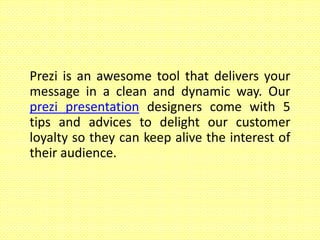The image features a light yellow background, reminiscent of a Post-it note, with black text centrally aligned. The text states: "Prezi is an awesome tool that delivers your message in a clean and dynamic way. Our Prezi presentation designers come with five tips and advice to delight our customer loyalty so they can keep alive the interest of their audience." Notably, the phrase "Prezi presentation designers" is highlighted in blue and serves as a hyperlink. The text comprises six lines and occupies roughly the middle third of the image. The font is justified, ensuring equal margins on both the left and right sides.